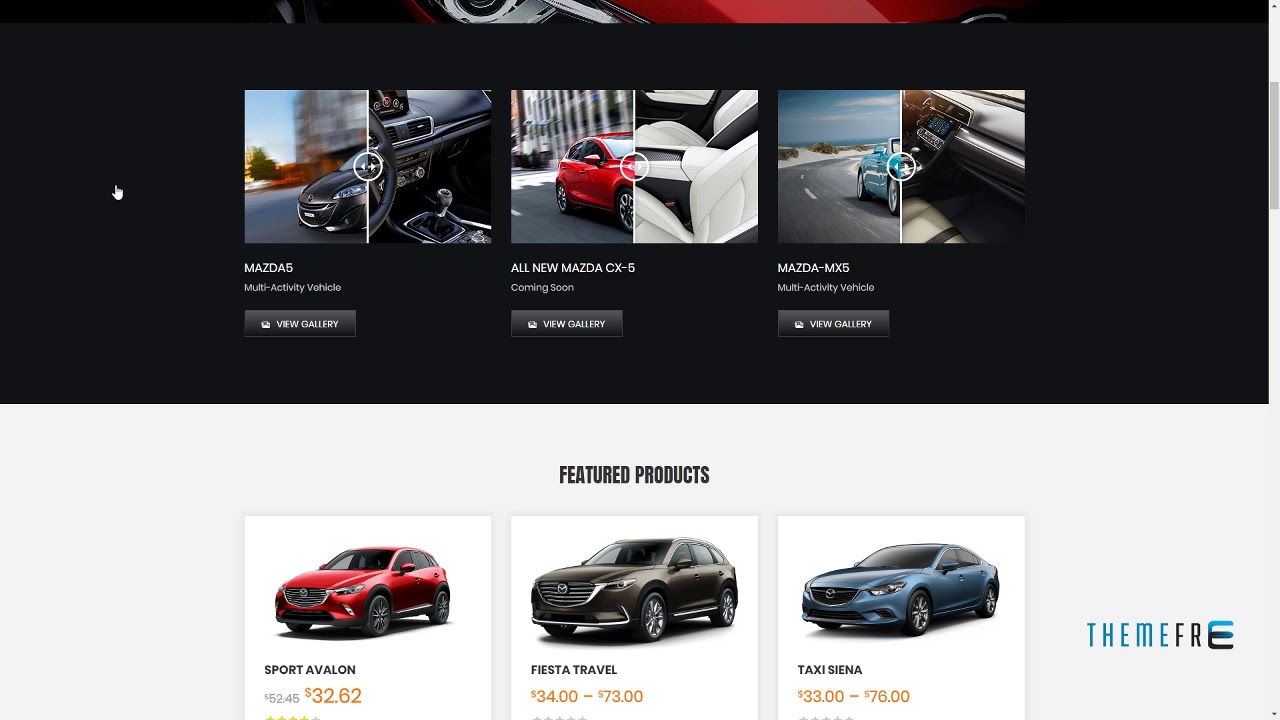The webpage showcases a striking Mazda promotion. The top half features a sleek black background, highlighting the bottom edge of a car with a vibrant candy apple red paint job and gleaming chrome trim. Below this, three images are displayed side-by-side, each presenting a different Mazda vehicle.

The first image features a black Mazda 5 multi-activity vehicle on a black asphalt road at sunset. The backdrop includes an apartment-style building and distant trees. The interior of this vehicle is shown to be elegantly outfitted in all black leather.

The second image introduces the all-new Mazda CX-5, which is set to be released soon. This car boasts a rich red exterior with chrome hubcaps, while its interior showcases a sophisticated blend of white and gray leather seats.

In the third image, a sky-blue Mazda MX-5 convertible is seen driving on a scenic beach highway, flanked by white sand. The sky above is clear and blue, and the road beneath is pristine black asphalt. The interior of the MX-5 features stylish gray leather seats.

Complementing these images, the bottom section of the webpage shifts to an off-white background and displays three additional vehicles. The first is a vibrant red Sport Evalon, followed by a bronze Fiesta Travel, and finally, a blue Taxi Sienna.